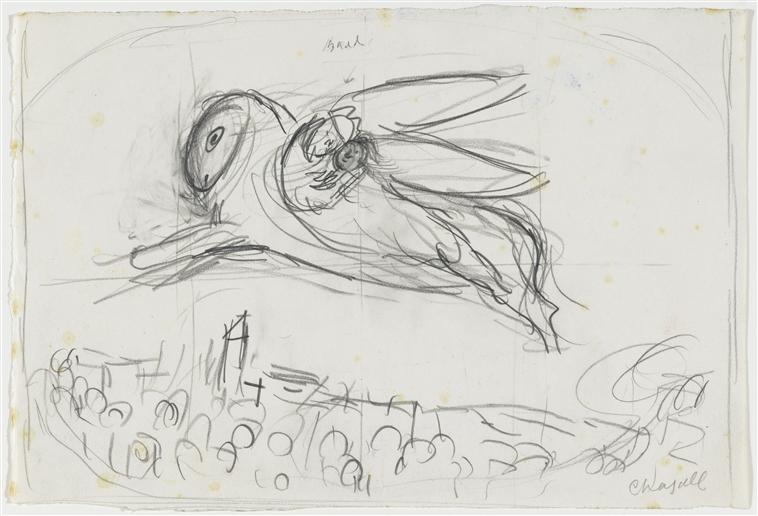This image is a pencil sketch of a large, winged, mythological creature with four legs, combining features reminiscent of an owl's face and a rabbit's body. The creature, which has an eye but no other facial features, appears to be either leaping or flying. Atop the creature's back are two small, faceless figures hugging each other. The detailed background below depicts a simple, scribbled portrayal of a small village with arched-roof homes, a river, cemetery stones, and a steeple topped with a cross. The art, possibly drawn by a child, is rendered in black, white, and gray on slightly yellowed paper, with quick, simple lines. The artist's name, which appears to be "Chagall" or "Chasell," is marked in the bottom corner.